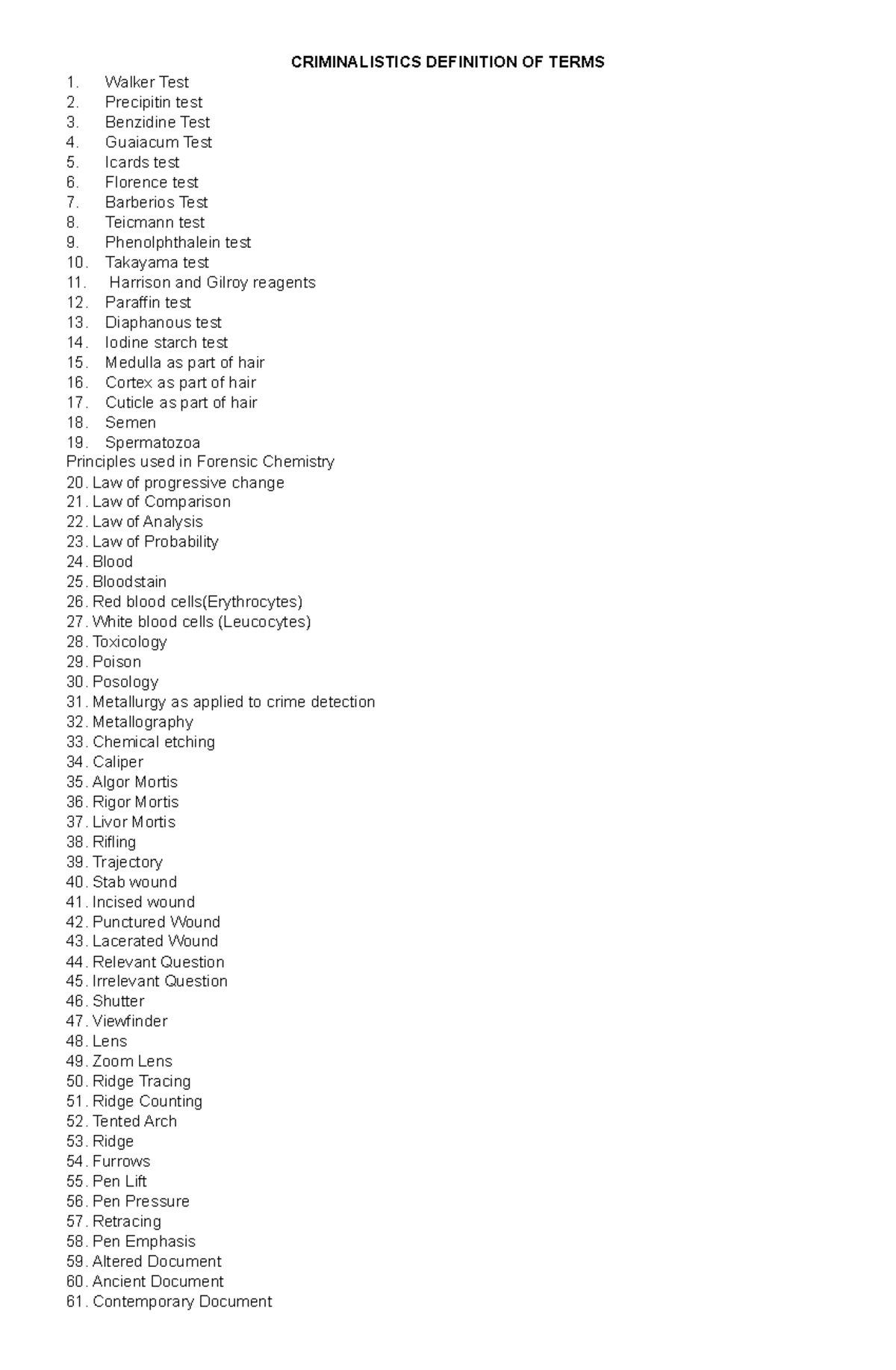This image features a meticulously categorized list titled "Criminalistics Definition of Terms." Despite lacking actual definitions, it enumerates various terms applicable in the field of forensic science, each associated with specific tests, principles, or elements of criminal investigation. The list is structured sequentially from numbers 1 to 61, encompassing a wide range of forensic concepts:

1. **Walker Test**
2. **Precipitant Test**
3. **Benzidine Test**
4. **Puiacum Test** (spelled P-U-A-I-A-C-U-M)
5. **Icards Test**
6. **Florence Test**
7. **Barbarios Test**
8. **Teichmann Test** (spelled T-E-I-C-H-M-A-N-N)
9. **Phenolphthalein Test**
10. **Takayama Test**
11. **Harrison and Gilroy Reagents**
12. **Paraffin Test**
13. **Diaphanous Test**
14. **Iodine Starch Test**
15. **Medulla as Part of Hair**
16. **Cortex as Part of Hair**
17. **Cuticle as Part of Hair**
18. **Semen**
19. **Spermatozoa**
20. **Principles used in Forensic Chemistry:**
    - **Law of Progressive Change**
    - **Law of Comparison**
    - **Law of Analysis**
    - **Law of Probability**
21. **Blood**
22. **Blood Stain**
23. **Red Blood Cells** (Erythrocytes)
24. **White Blood Cells** (Incorrectly listed as Erythrocytes again)
25. **Toxicology**
26. **Poison**
27. **Posology**
28. **Metallurgy as Applied to Crime Detection**
29. **Metallography**
30. **Chemical Etching**
31. **Caliper**
32. **Algor Mortis**
33. **Rigor Mortis**
34. **Liver Mortis**
35. **Rifling**
36. **Trajectory**
37. **Stab Wound**
38. **Incised Wound**
39. **Punctured Wound**
40. **Lacerated Wound**
41. **Relevant Question**
42. **Irrelevant Question**
43. **Shutter**
44. **Viewfinder**
45. **Lens**
46. **Zoom Lens**
47. **Ridge Tracing**
48. **Ridge Counting**
49. **Tented Arch**
50. **Ridge**
51. **Furrows**
52. **Pen Lift**
53. **Pen Pressure**
54. **Retracing**
55. **Pen Emphasis**
56. **Altered Document**
57. **Ancient Document**
58. **Contemporary Document**

This extensive compilation showcases the diverse spectra of terms integral to criminalistics, underscoring the breadth of tests, forensic techniques, and scientific principles employed in the intricate investigation of criminal cases.